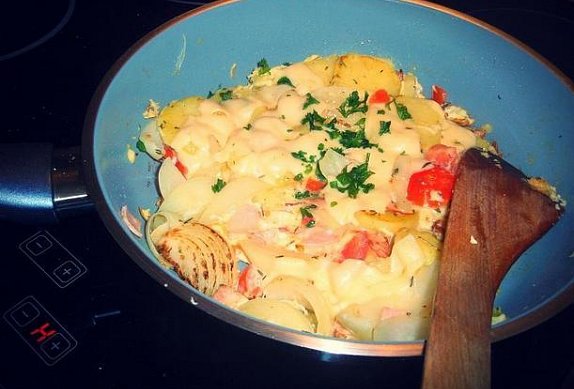In the image, a vibrant blue skillet with a matching blue handle and inner lining rests on a black, flat-top stove surface that suggests a kitchen setting. Ensconced within the skillet is a mixture of food featuring oval-shaped noodles, diced tomatoes, chopped onions, and possibly cilantro or parsley, complemented by a pale yellow, translucent cheese, lending a possible indication of a potato-based or pasta dish. The meal appears either fully or nearly ready to be cooked, as evidenced by the wooden stirring utensil with a flat end placed inside, poised for blending the ingredients. The scene's colors, including blue, black, gold, yellow, red, orange, brown, and white, enhance the depiction of a cozy, homely environment focused on a culinary creation.